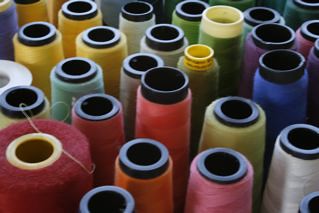The image showcases an array of vibrantly colored industrial-strength spools of thread closely grouped together, resembling what might be found in a carpet mill. The scene highlights a diverse palette with dominant colors including several shades of yellow, pink, and white. On the left side, there are four yellow spools clustered, while additional colors such as blue, green, purple, and a unique light teal are interspersed throughout. Among the assortment, one particularly large spool stands out in the lower area of the image. The spools rest on black plastic bases, except for three distinct spools. Though the view doesn't allow for a full display, approximately 15 spools are visible from the top in this detailed close-up, capturing the spectrum of hues against a black background.